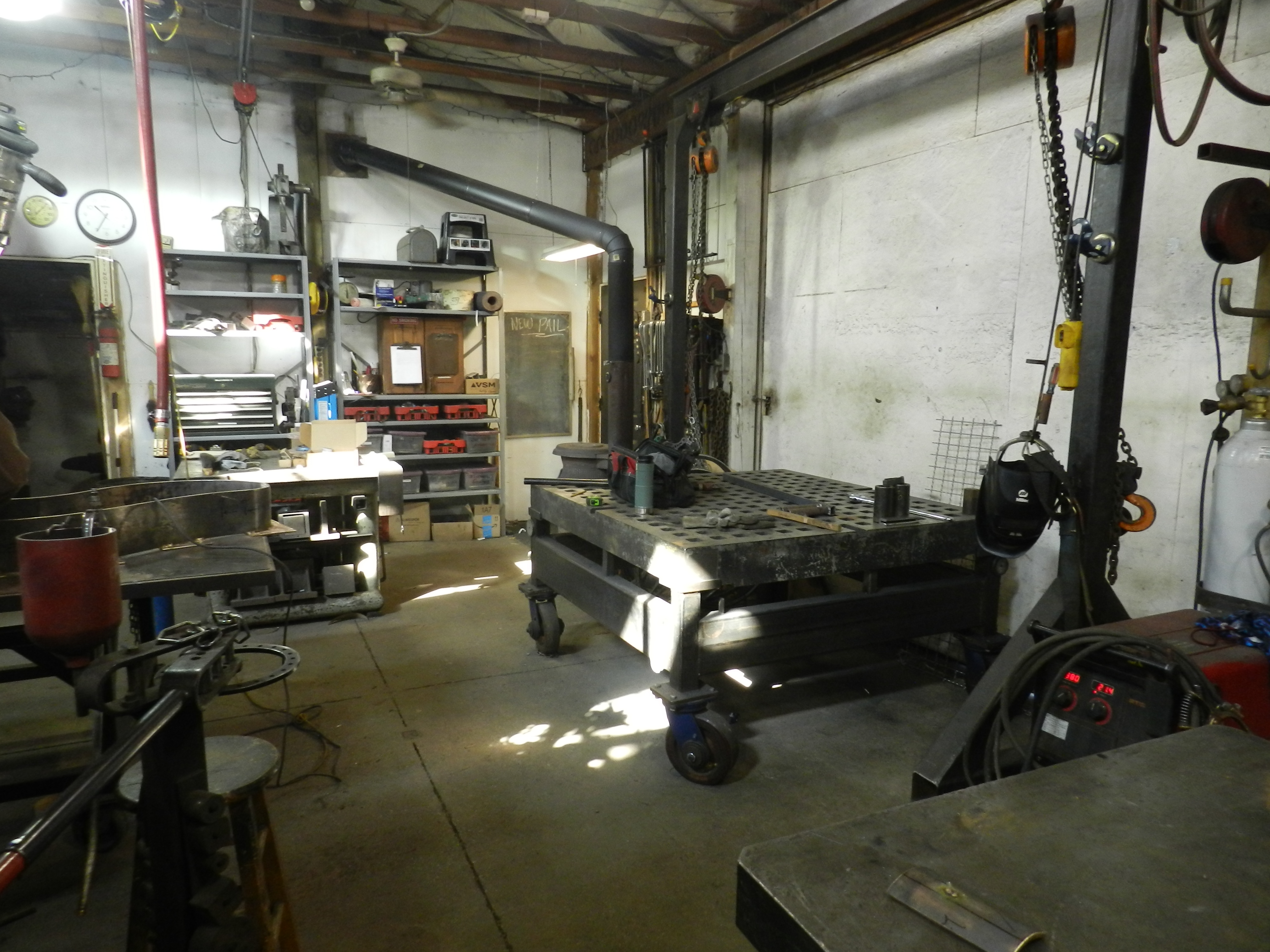The image depicts a detailed view of an industrial-looking workroom, likely a garage or basement. The space features concrete floors and slightly dirty white walls, heavily occupied with various metal contraptions, tools, and equipment. Prominently in the foreground to the bottom right, there is a metal stand and a metal machine, with another metal stand equipped with wheels beside it. A black pipe extends from one of these machines to the wall, hinting at a connection to a furnace or possibly a wood stove, as a furnace pipe is visible. Additionally, other notable items include a giant lift, a generator, an iron table, and a welding machine. An assortment of tools and equipment is distributed around the room, lying on shelves and workstations, including a stool and a jack. The back wall of the room features shelving filled with tools, a clock, and a black chalkboard with indistinct writing, possibly "New Pale" or "Paul". Steel beams stretch across the room up to the rafters, indicating a sturdy, industrial structure. This work area appears well-used, functional, and filled with the essentials for a variety of mechanical or industrial tasks.